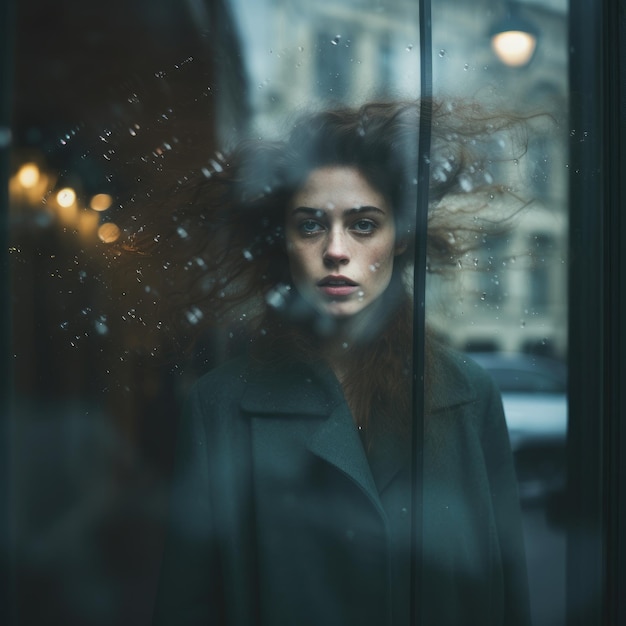The image depicts a professional photograph or possibly a movie scene of a light-skinned young woman with wide-open eyes, giving her an expression of fright or intense focus. She stands at the center, looking straight ahead, possibly through a rain-streaked window, as raindrops create blurred spots on the glass. Her long, dark, stringy hair blows dramatically to the right, suggesting a strong wind. She is dressed in a dark blue-black overcoat, with hints of a red shirt visible underneath. The background features an out-of-focus off-white building and faint reflections of streetlights creating little orange and white orbs, with a distinct streetlight hanging in the upper right corner. The left side of the image has a dark shade with an orange hue intermingling, possibly from additional streetlights or ambient reflections. The scene suggests a rainy street view at night, with the woman potentially separated from the viewer by the windowpane.